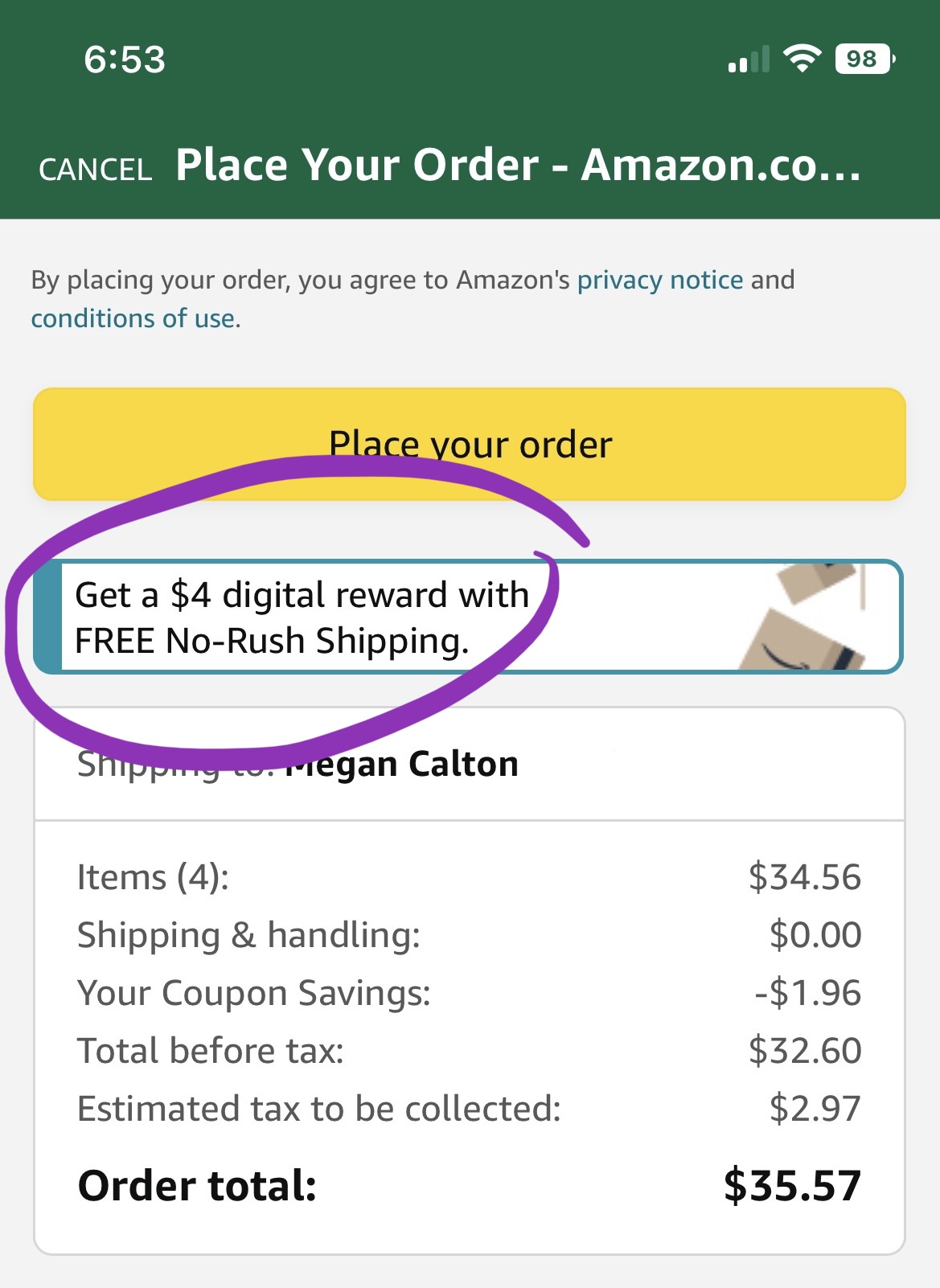The image showcases a screenshot from a Selfonore tablet displaying an Amazon purchase page. At the very top, a wide strip of dark olive green features the number "653" in white on the left, and on the right, indicators for network signal (2 out of 4 bars), full Wi-Fi signal, and a 98% battery level. 

Just below, within the green strip, the word "Cancel" appears as an option, followed by the bold, larger font phrase: "Place Your Order - Amazon.co...". Underneath, it states, "By placing your order, you agree to Amazon's Privacy Notice and Conditions of Use."

Further down, a prominent yellow button with black text reads "Place your order." A small purple-circled banner advertises, "Get a $4 digital reward with free No-Rush Shipping." 

The order details follow: 
- "Shipping to Megan Colton"
- "Items Total: $34.56"
- "Shipping & Handling: $0"
- "Coupon Savings: -$1.96"
- "Total Before Tax: $32.60"
- "Estimated Tax: $2.97"

The final "Order Total" amounts to $35.57.